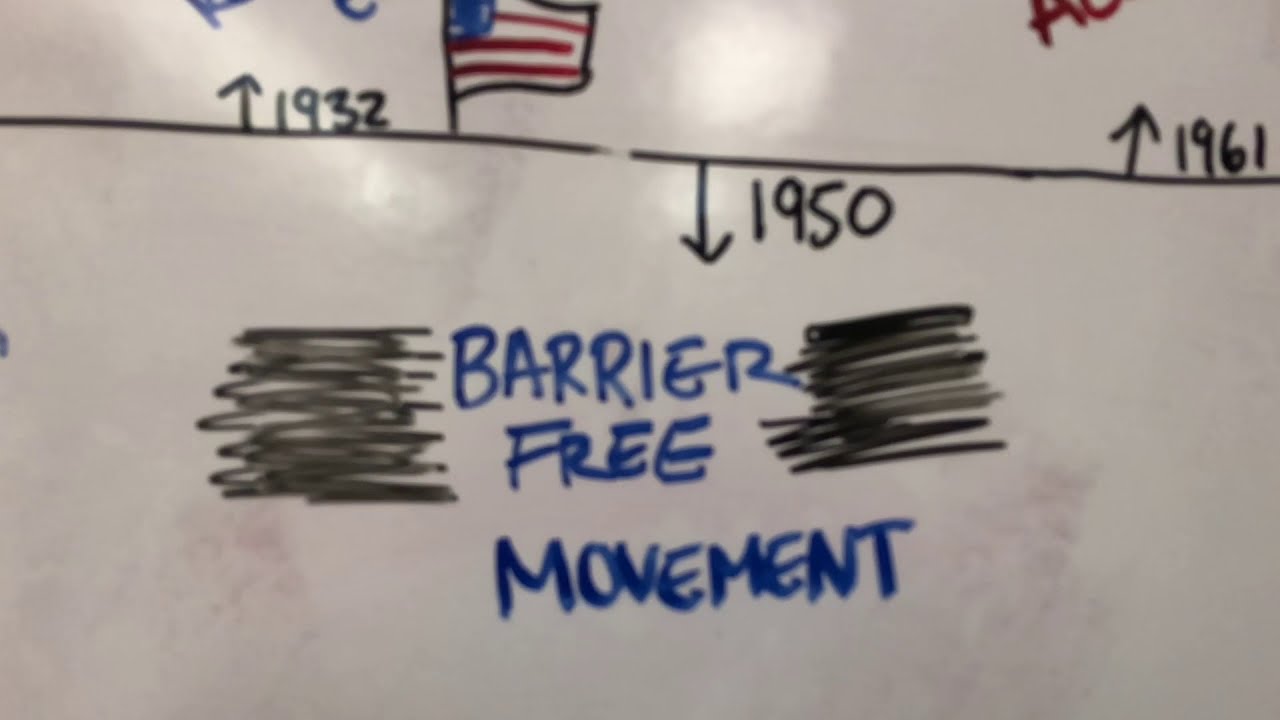The image depicts a rectangular, close-up view of an aged whiteboard with various marker drawings and text. At the top third to fourth of the whiteboard, there is a horizontal black line that starts about an inch from the left edge and extends almost to mid-center before breaking briefly and continuing to the far right side. On the left end of the black line, a black arrow points upwards with the number '1932' next to it. Adjacent to this date is a small drawing of an American flag, characterized by red and white stripes and a blue square in the top left corner.

In the center of the black line, there is an arrow pointing downwards with the date '1950'. This arrow directs attention to the phrase "barrier-free movement" written in bold, dark blue letters in the middle of the whiteboard. To emphasize the message, there are horizontal black squiggly lines flanking the text "barrier free" on both the left and right sides.

Further to the right on the black line, there is another upward-pointing arrow annotated with the date '1961'. At the extreme right edge of the photo, partially cut off, is a red letter 'A'.